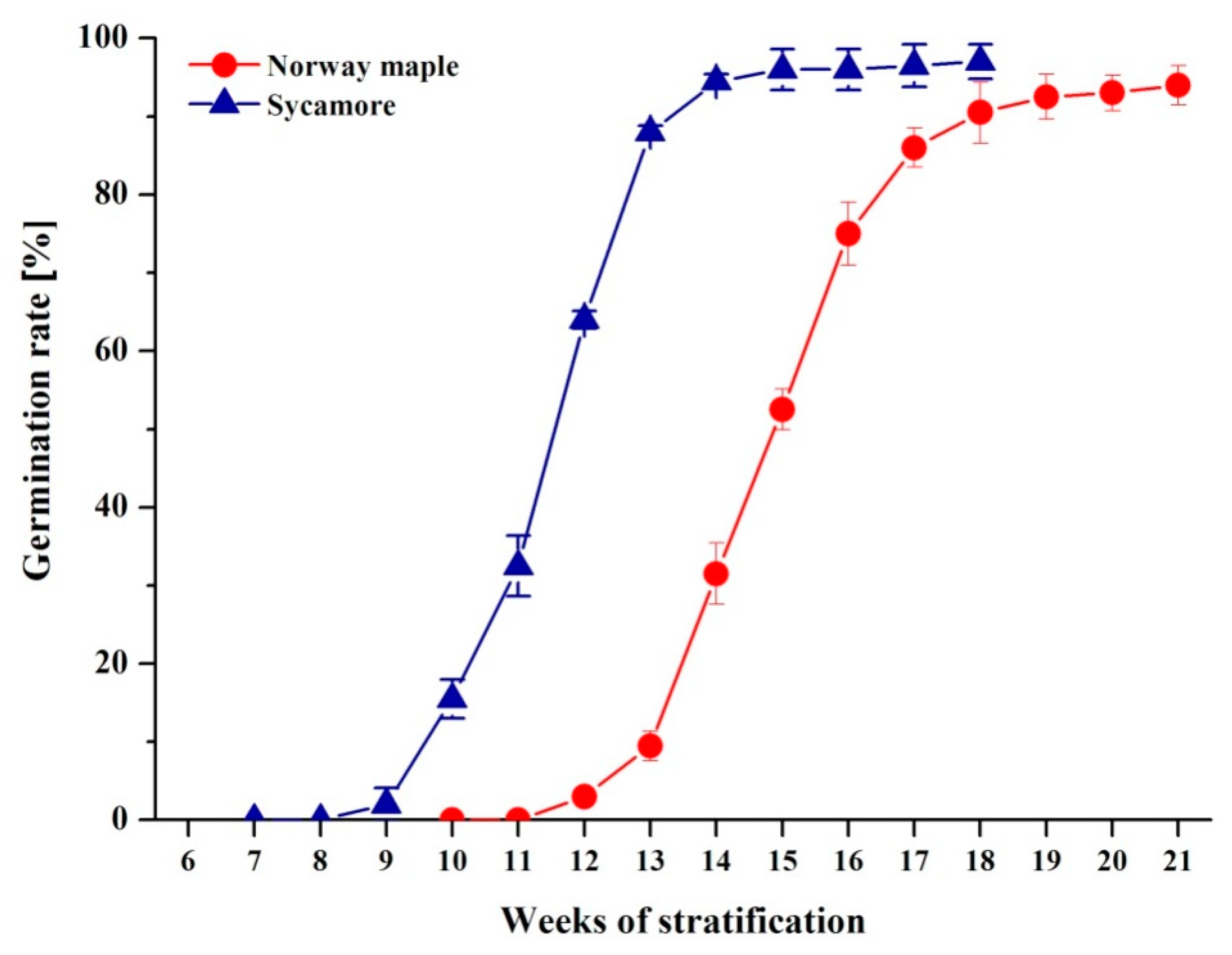The image is a line graph with a white background, depicting germination rates of Norway Maple and Sycamore trees over a period of weeks of stratification. The x-axis, labeled "Weeks of Stratification," ranges incrementally from 6 to 21, while the y-axis, labeled "Germination Rate (%)", ranges from 0 to 100% in 20% intervals with additional markings at 10, 30, 50, 70, and 90. The graph features two distinct curves: a blue line marked with triangles representing the Sycamore on the left, and a red line marked with circles representing the Norway Maple on the right. The key at the top indicates these representations, with red circles for Norway Maple and blue triangles for Sycamore, illustrating the germination rates corresponding to the weeks of stratification.